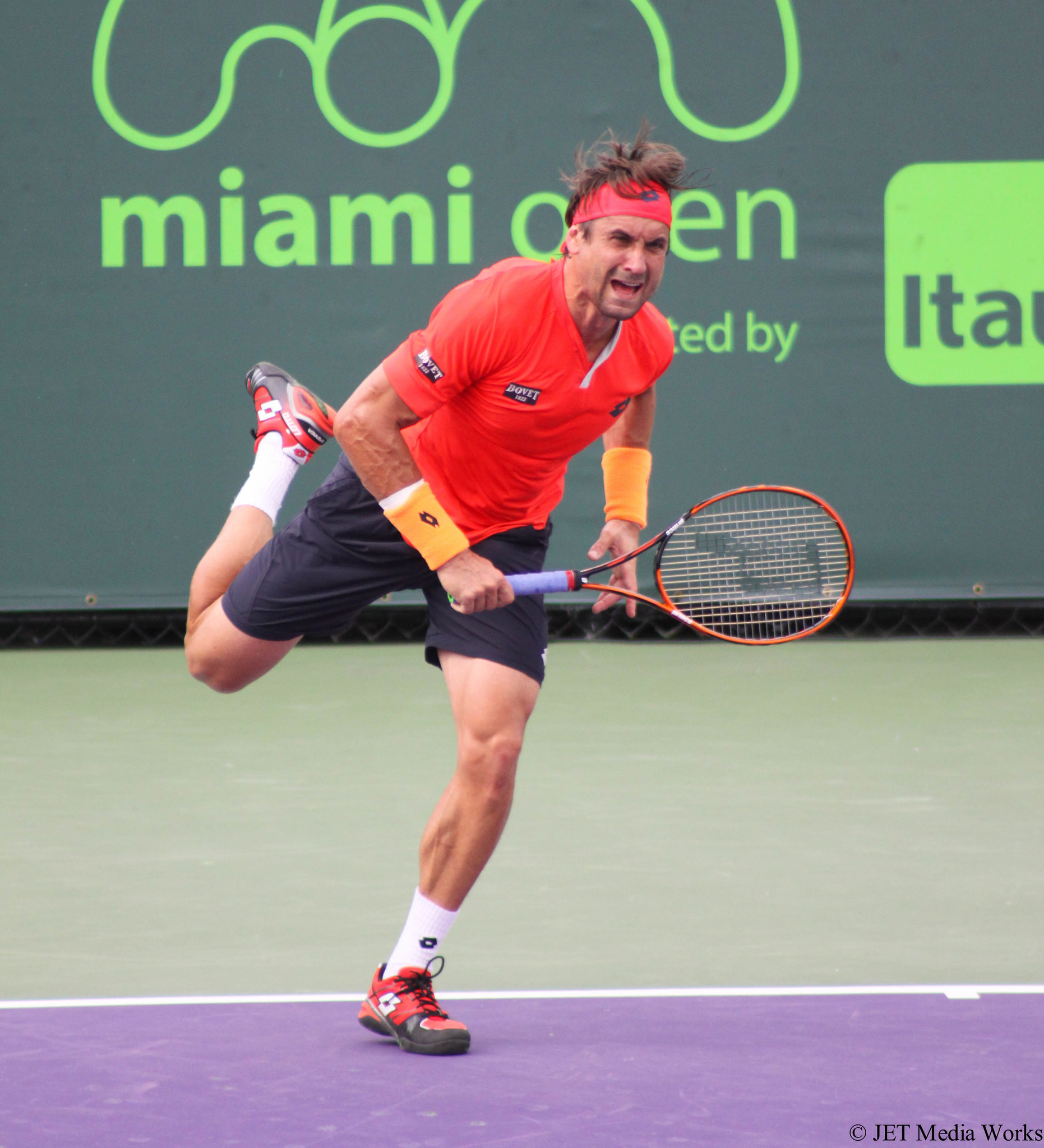In the image, a tennis player, who resembles Andre Agassi, is prominently featured at the center of the scene, playing on a tennis court. The court has a distinctive purple surface with painted lines, indicative of a possibly hard clay or hard flooring typical of professional tennis courts. The setting is outdoors, likely midday, as suggested by the bright lighting.

The athlete is dressed in a red shirt and matching red headband, through which his hair sticks out wildly. He also wears red shoes with a black stripe, white socks, and appears very muscular. His right foot is bent up nearly touching his backside, indicating a dynamic and active stance as he leans toward his right side, gripping a tennis racket with a blue handle and an orange border.

In the background, the wall features text partially obscured by the player's body, but it reads "Miami Open" with additional circles in green. The ground surface is segmented: purple where the player stands and green further back in the court. Finally, the image bears a copyright indication at the bottom that reads "Jet Media Works." The colors evident in the scene include purple, white, olive, black, tan, red, orange, green, and light green.